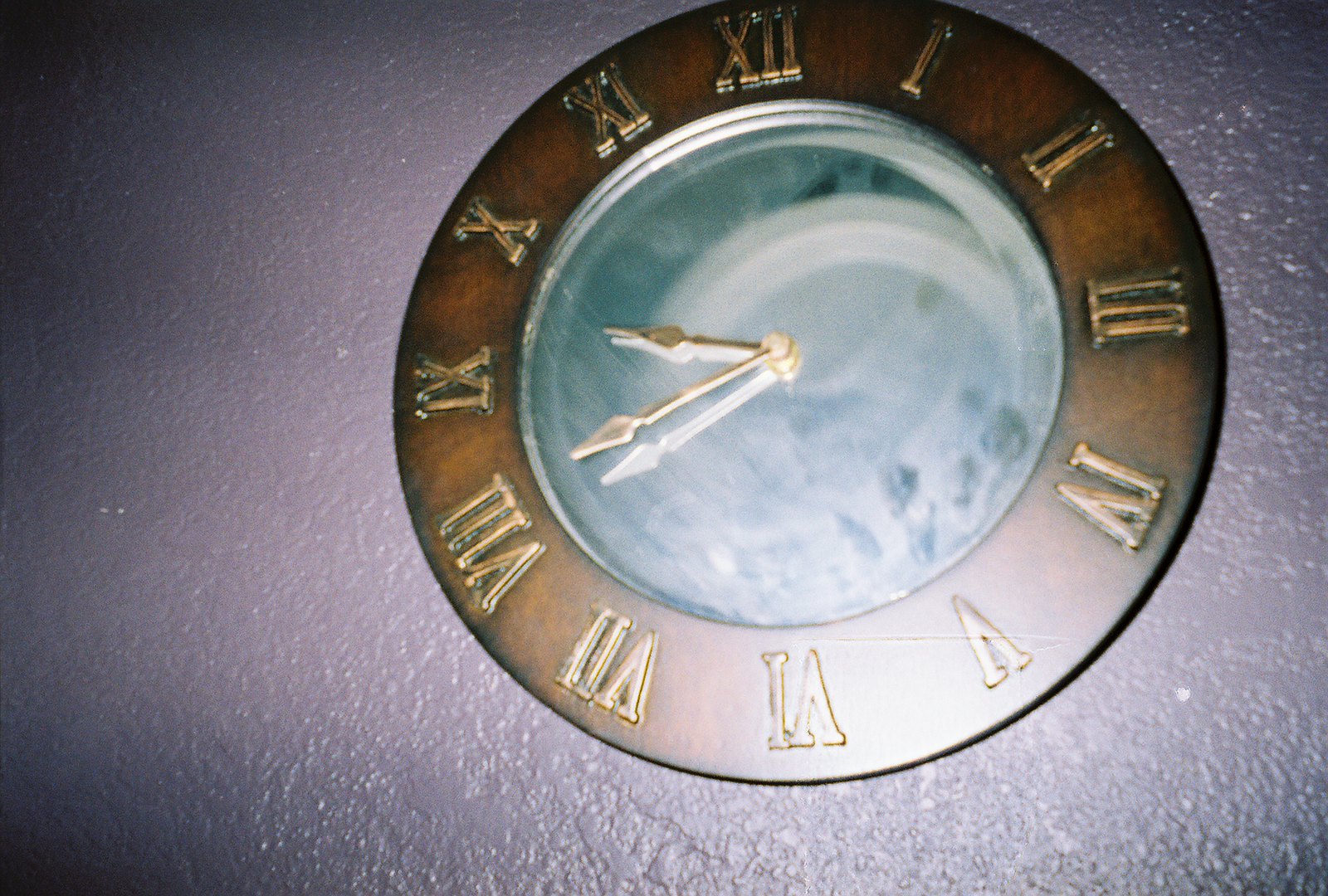A thin metallic clock is mounted on a textured, dark brown stucco wall, adding a touch of elegance to the setting. The clock face is made of a glossy, reflective material, which adds sophistication and shine. Uniquely, it features no modern numbers; instead, it displays classic Roman numerals in a gold-tone bronze that matches the brass-colored minute and hour hands. The outer edge of the clock is wide and coated in a rich, antique brown finish, providing a striking contrast to the reflective clock face. The hands of the clock indicate the time as 20 minutes to 10.